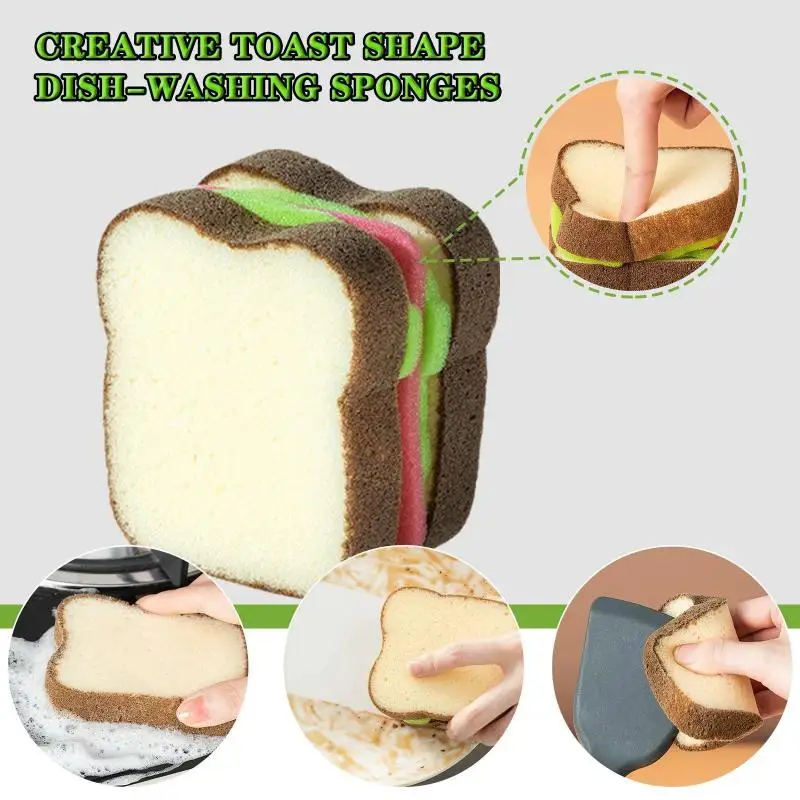The advertisement showcases the Creative Toast Shaped Dishwashing Sponges against a light grey background. Prominently at the top, in bold green text, it reads "Creative Toast Shaped Dishwashing Sponges." The featured product is a whimsical kitchen sponge designed to resemble a sandwich. The sponge has two pieces of white bread with a dark brown crust, while the inside layers consist of pink and green sponge material, mimicking slices of meat and lettuce. An eye-catching circle with dashes highlights a close-up of a finger pressing down on the sponge, demonstrating its softness. At the bottom, three smaller circular images illustrate the sponge in action: one shows it lathered with soap cleaning a stove, another depicts it wiping down a white countertop with a brown stain, and the last image highlights the sponge cleaning a spatula.